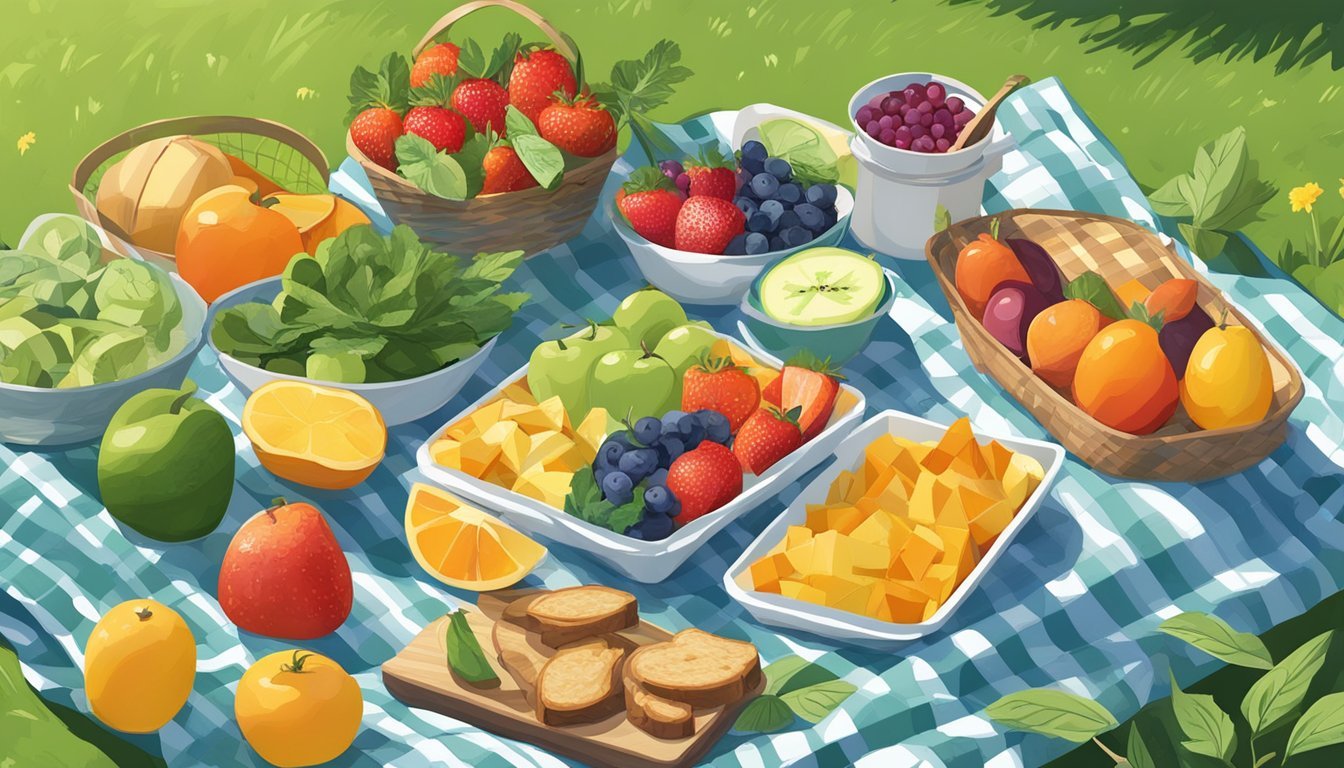The hand-drawn illustration captures an inviting picnic scene set outdoors. Spread out on a green and white checkered blanket, which is laid on a vibrant green grassy patch, is an assortment of appetizing food items. At the center of the blanket, there's a white tray filled with an assortment of fruits, including green apples, blueberries, strawberries, and mangoes, some of which are already cut. Adjacent to it sits a square tray with yellow fruit, and next to the centerpiece is a cutting board topped with brown bread.

On the lower left, there's a cutting table with additional bread, while the upper part of the blanket features various bowls and wicker baskets filled with colorful items. A white bowl overflows with strawberries and blueberries, and another wicker basket holds red strawberries. There are also jars of raspberry compote and an additional wicker basket containing orange-yellow fruits. The picturesque setup is completed with bowls of salads, including leafy greens and sliced oranges and apples. The right side of the image is highlighted with a few green leaves and a bright yellow flower, adding a touch of nature's charm to this delightful picnic illustration.